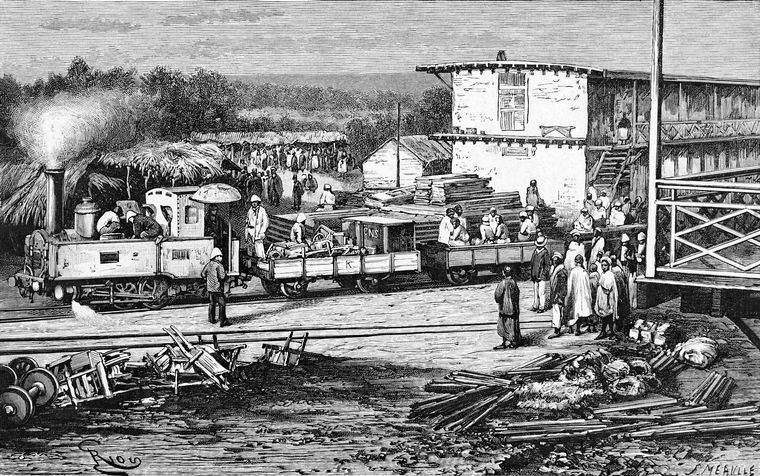This black-and-white illustration, potentially a charcoal sketch, depicts a bustling scene from what appears to be the 1800s. Dominating the center, a small, uncovered steam engine moves from right to left, trailing several short, loaded carts. The engine emits a large billowing cloud of gray smoke from its smokestack. The tracks, newly constructed, have debris such as logs and broken furniture scattered beside them.

The train transports numerous laborers, all wearing hats, and a single operator is visible. Groups of onlookers, including what might be a supervisor or officer, are gathered around, observing the activity. A long, thin, two-story wooden building with white siding, which could be a hotel or barracks, stands prominently in the background on the right. The scene is animated and vibrant, with some structures resembling a marketplace further enriching the backdrop.